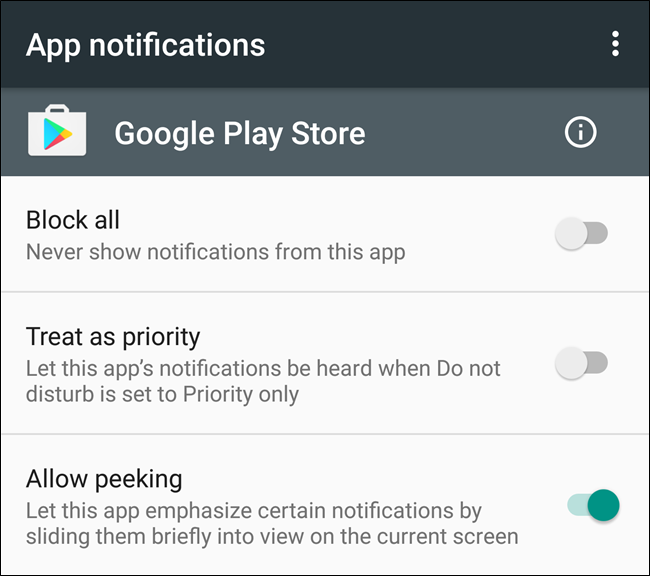The image depicts a notification settings screen for an Android device, specifically for the Google Play Store app. The top section of the interface displays "App Notification" against a black background, with an ellipsis icon on the right side, indicating additional options. Below this, there is a dark gray box featuring a white bag icon with the Google Play symbol in the center. Next to the icon, it says "Google Play Store," and a circular icon with a lowercase 'i' in the middle is displayed, suggesting information or settings details.

Underneath this section, there are three white rectangles with different notification settings. The first rectangle reads "Block all," with a description stating, "Never show notifications from this app." The toggle bar next to it is gray and turned to the left, indicating that this option is disabled. The second rectangle is labeled "Treat as priority," explaining, "Let this app's notifications be heard when Do Not Disturb is set to Priority only." This toggle bar is also gray and turned to the left, showing it is disabled. The final rectangle says "Allow peeking," which means, "Let this app emphasize certain notifications by sliding them briefly into view on the current screen." The toggle bar for this setting is turned to the right and colored a greenish-turquoise hue, signifying that the option is enabled.